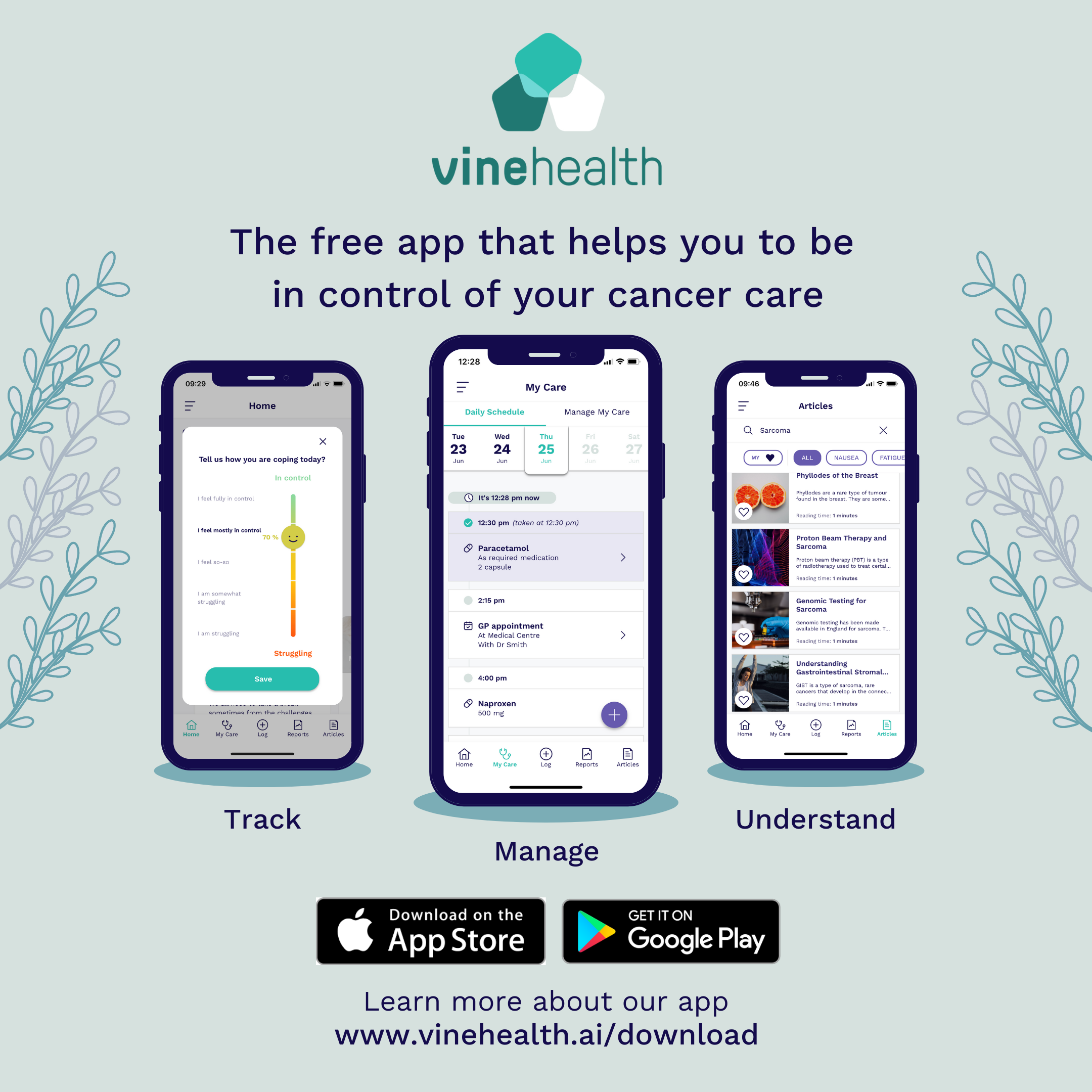This image appears to be an advertisement for Vine Health, featuring their emblem, which consists of three interconnected pentagons. The pentagons vary in color, with one being deep teal, another slightly lighter teal, and the last one a translucent white. The text next to the emblem reads, "Vine Health - The free app that helps you to be in control of your cancer care."

The advertisement prominently displays three smartphones. The central phone is the largest and emphasizes the app's features. At the top, the word "Track" is displayed, followed by the prompt, "Tell us how you are coping today." To the left of the prompt, a vertical progress bar starts from "Struggling" at the bottom and ends with "In Control" at the top. On this particular example, a smiley face icon is positioned at 70% in the yellow zone, indicating the user's current state, with a label stating, "I feel mostly in control." Below the yellow zone, additional markers read, "I feel so-so," followed by, "I'm somewhat struggling," and, at the bottom, "I am struggling."

The next section of the central phone displays a medication reminder, stating, "12:30 PM, Para-actomo." This area highlights the app's "Manage" feature, helping users keep track of their medication schedules.

The third phone on the right features the text "Understand," rounding out the application's core functions to help users track, manage, and understand their cancer care.